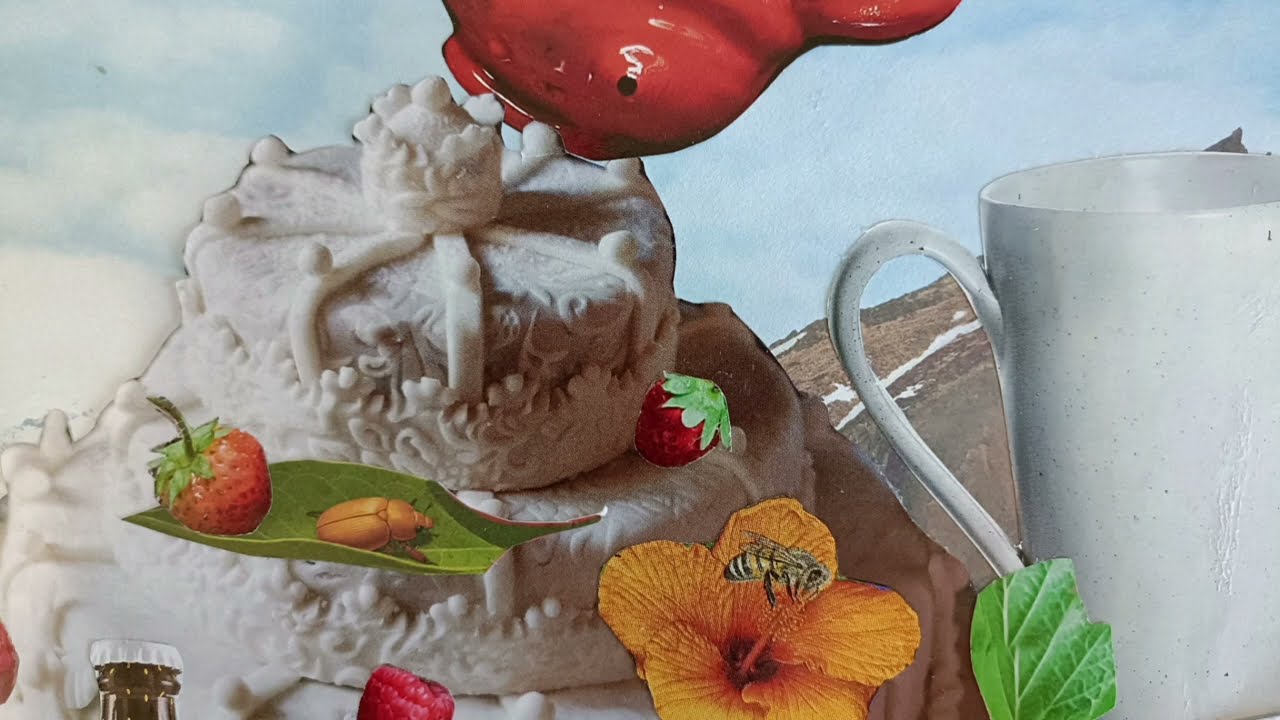The image features a detailed, white multi-tiered cake, possibly a wedding cake, intricately decorated with ornate designs. An orange hibiscus flower with a bee nestled in its stamen adds a colorful touch atop the cake. Accompanying the cake is a green leaf bearing a strawberry and a small beetle. A plain white mug appears on the right side of the image, with another small leaf at its base. The backdrop is a vivid blue sky adorned with white clouds and hints of a mountainous landscape. Additional elements include a yellow flower with a bee and a bottle with a white cap. The entire composition is colorful yet predominantly white, giving it an almost animated or composite appearance.